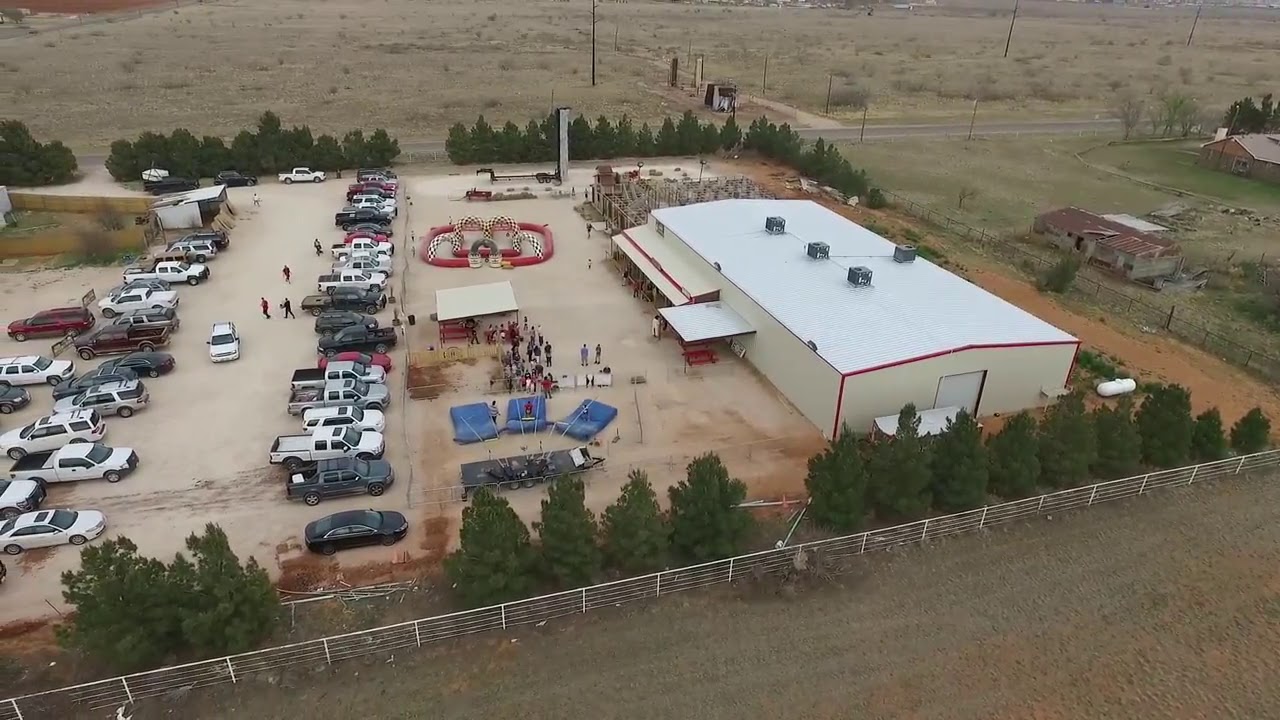This aerial photograph captures a bustling scene centered around a large, cream-colored garage with red trim and a white, sloped roof adorned with several air conditioning units. The rectangular building, possibly acting as a business or flea market, features a prominent closed white door at the front. Adjacent to the garage are sections shaded by light yellow awnings with red stripes, and below these, a light gray square is affixed to the side of the building.

The expansive, dirt parking lot surrounding the garage is teeming with activity. Lined with rows of various vehicles – including black, green, white, and silver cars and trucks – the lot is interspersed with groups of people milling about. Toward the left, the parking is less organized, with vehicles parked haphazardly. In the center, a distinct play area boasts a variety of children’s entertainment, including a bouncy structure and blue mattress-type attractions, suggesting a family-friendly environment which might include a petting zoo given the hay bales and small barn area.

Encircling the lot is a sturdy white metal fence, accompanied by dense rows of evergreen trees that provide a natural barrier before stretching out into vast farm fields. In the distance, there is a weathered shed with a brown roof and green walls, giving the appearance of abandonment amidst the desert-like, brown and yellow grass landscape. Power poles punctuate the terrain, and a few structures hint at habitation, including an adjacent house. This dynamic and multi-functional area blends commercial and recreational spaces harmoniously within a rustic, rural setting.